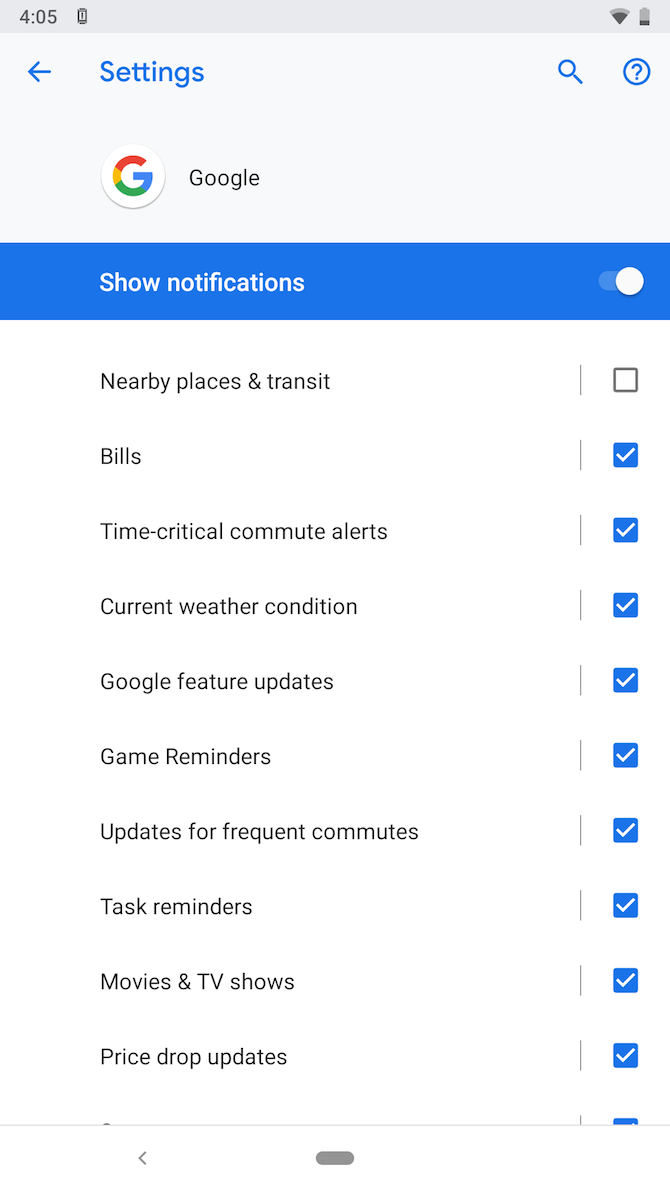This is a screenshot of a Google settings page taken from someone's phone at 4:05. At the top of the image, "Settings" is displayed in blue with a left-pointing arrow beside it. Below this, the Google symbol with its distinctive multicolored "G" (red, yellow, green, and blue) is prominently featured. The settings page is organized to manage notifications for various categories.

A blue banner at the top of the page reads "Show notifications," accompanied by a toggle switch to turn notifications on or off. The listed categories for notifications included nearby places and transit, bills, time-critical alerts, commute alerts, and current weather conditions. Each category has a corresponding checkbox on the right; all checkboxes are marked, except for the "Nearby places and transits" option, which remains unchecked. The checkboxes themselves are blue, indicating which categories have active notifications.